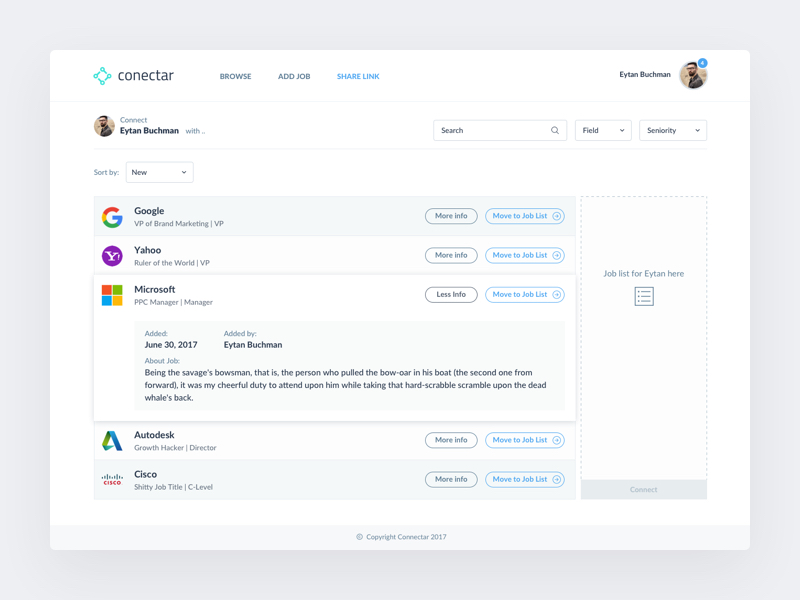The image depicts a user interface with a gray border surrounding a white central area. In the top left corner, there's a light blue section that includes the words "Connect" or "ConnectAr," though it's unclear due to blurriness. Below this area, the interface has tabs or options labeled "Browse," "Add Job," "Share," and "Link."

On the main part of the screen, it appears there's a list of job listings or profiles. The top section shows various filtering options, including a search box, a field labeled "Field" with a drop-down button, and another labeled "Seniority." Additionally, there's a sorting option that allows the user to sort by "New."

The first job listing mentions a "Google VP of Brand Marketing" role with an associated button labeled "More Info" and another one labeled "Move to Job List." Below that, there's a listing for a "Yahoo Ruler of the World VP" position. The next listing mentions "Microsoft PPC Manager," with the date added being June 30, 2017, and an annotation "Added by Ethan Bushman." At the bottom of this section, there's an "About Job" label providing more detailed information about the job roles.

Overall, the text and interface elements are quite blurred, making it challenging to discern some details clearly.